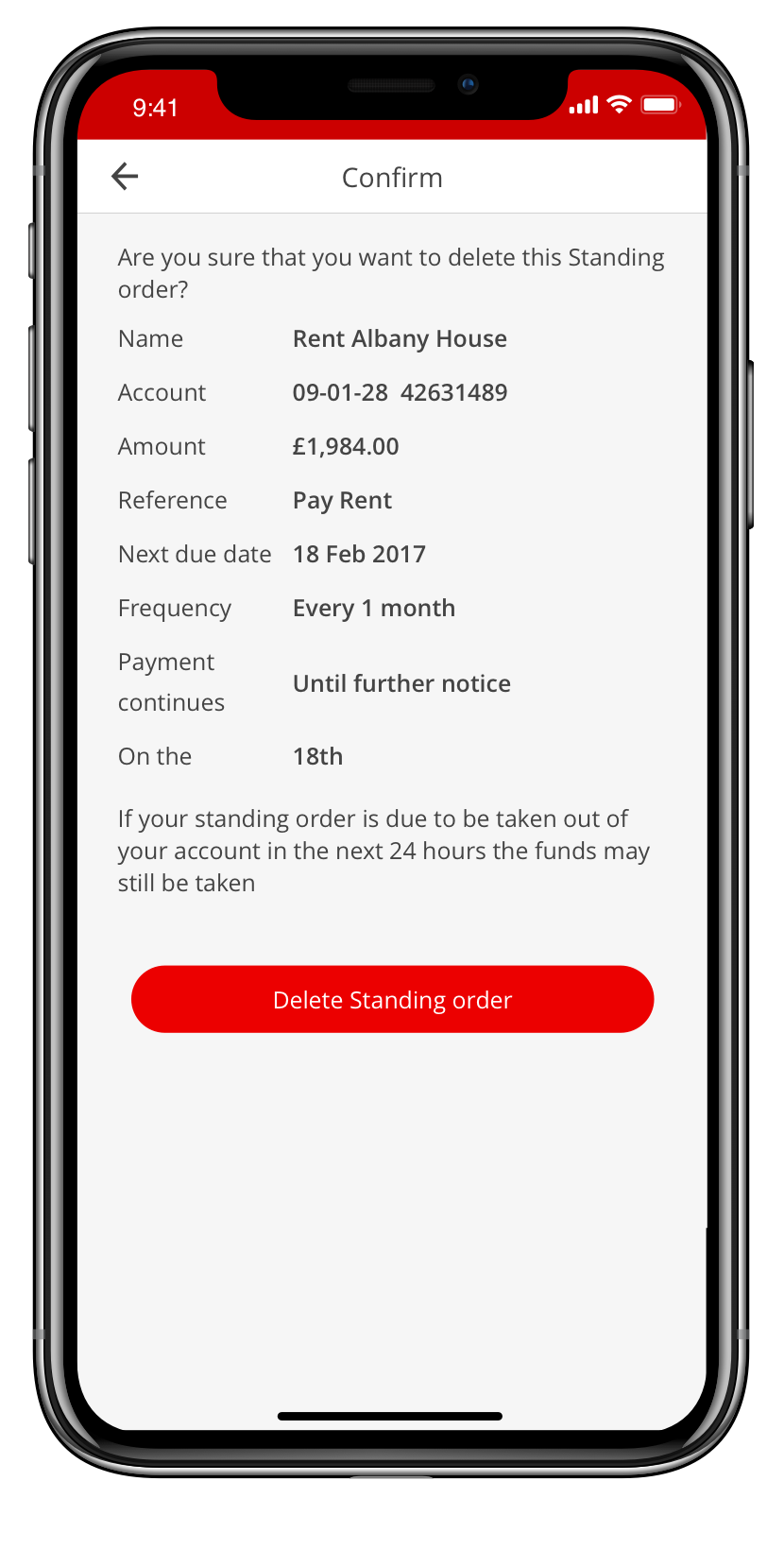The image is a screenshot of a smartphone displaying a confirmation prompt for deleting a standing order. The phone's status bar at the top right shows the time, 9:41, signal bars, Wi-Fi indicator, and battery status. The volume keys are visible on the left side of the phone, while the power button is on the right.

The main content of the screen asks, "Are you sure you want to delete this standing order?" Details of the standing order are provided:
- Name: Rent, Albany House
- Account Number: 09012842631489
- Amount: £1984
- Reference: Pay Rent
- Next Due Date: 18 February 2017
- Frequency: Every one month
- Payment continues until further notice on the 18th.

A cautionary note mentions that if the standing order is due to be taken out of the account in the next 24 hours, the funds may still be withdrawn.

At the bottom of the prompt, there is a red button labeled "Delete Standing Order." The phone outline is black, and the background of the confirmation prompt is predominantly white, with red sections at the very top and bottom of the screen. A black line is also present at the bottom.